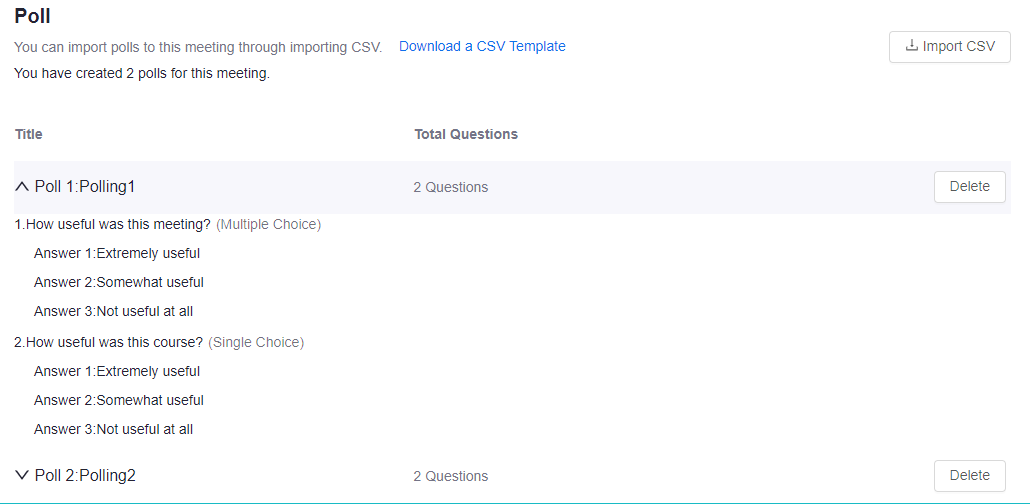The image features a user interface for importing and managing POE data. 

On the left side of the screen, set against a white background, is the capital letter "P" followed by the word "POE." Below, it reads "You can import POE," followed by the text "and upload CSV." To the right of this message, there is a blue button labeled "Download a CSV template."

On the right side, there is a gray-bordered rectangle with a white interior. Inside this rectangle, the text "Import CSV" is displayed in gray. Below this, in black text, it states, "You have created two POEs."

Following this statement is a section titled "POE1," written in black with "POE number one" in gray beneath it. The first question under this POE reads, "How useful was this meeting?" with the note "(multiple choice)" in gray. The multiple-choice answers are:
1. Extremely useful
2. Somewhat useful
3. Not useful at all

The second question asks, "How useful was this course?" with the note "(single choice)" in gray. The single-choice answers are:
1. Extremely useful
2. Somewhat useful
3. Not useful at all

Another section is titled "Polling2," followed by the note "two questions." Beneath this, there is a gray "Delete" button with a capital "D." The interface also shows the total questions for this section, which is noted as "Two questions" in gray. Each section is enclosed within a gray-outlined rectangle with a white interior.